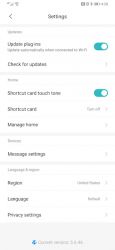This is a blurry screenshot of a mobile app's settings screen with a white background. At the top of the screen, the word "Settings" can be barely discerned, with a right-pointing arrow next to it. Directly below "Settings," there is an indistinguishable small black text on the left side. Further down, in bold black font, the text "Update Plugins" is visible, accompanied by a toggle switch to the right that is turned on and highlighted in blue. Below this, the phrase "Check for Updates" is also in bold, with a right-pointing arrow on its far-right side. The next section, marked by very small writing, begins with "Shortcut Card Touch" and another unreadable word along with another toggle switch that is similarly toggled on and highlighted in blue. At the bottom of this section, to the right, there appears to be text related to "Shortcuts Card, Manage" but it remains too blurry to read clearly. The screenshot terminates with a thick gray border at the bottom of the screen.